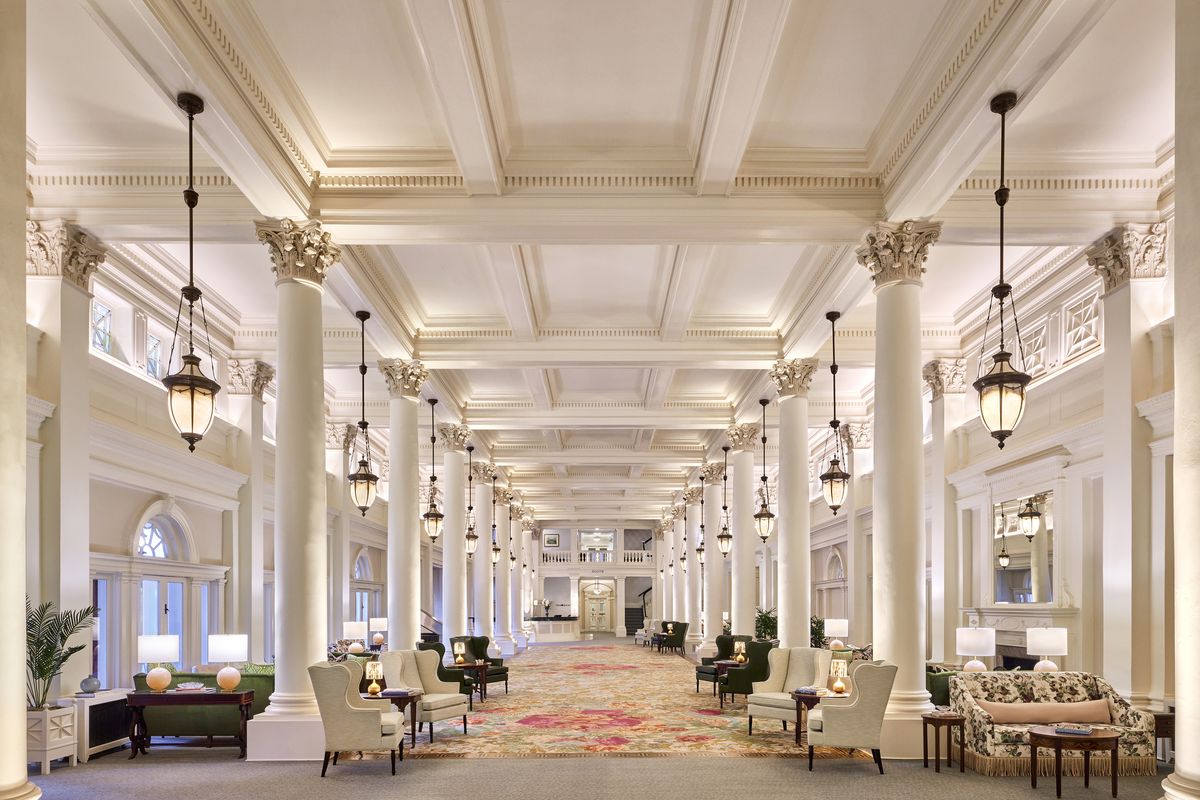The image portrays a lavish and expansive interior of what appears to be either a grand mansion or a luxurious hotel lobby. The room is adorned with numerous tall, white pillars that extend seemingly endlessly, creating an illusion of infinite space. These pillars feature intricate golden detailing at their capitals and are mirrored on either side by elegant, high-quality hanging lamps with brown bases attached to the white ceiling.

The floor is covered with a large, elaborate carpet featuring rows of light green, pink, and golden patterns. Cushioned chairs in white and green hues, along with matching long sofas, line the hall, emphasizing the room’s opulence and uniformity. Between these seating arrangements, brown tables bearing table lamps are positioned, adding to the grandeur.

The room's decor includes mirrors on one side and Norman-style window designs on the other, enhancing the sophisticated ambiance. Notably, at the far end of the hall, a balcony-like structure is visible, further contributing to the stately setting. The overall design suggests a space of significant importance, akin to prestigious buildings such as the White House.